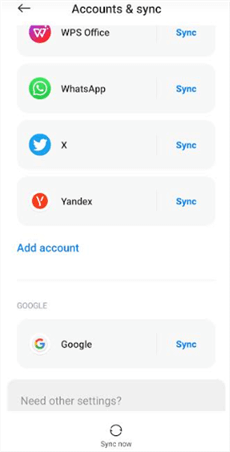This is a detailed screenshot captured from an Apple phone, featuring an "Accounts and Sync" settings page. The user interface displays several interactive elements aligned neatly in a minimalist and functional design.

At the top left corner, there's a gray arrow pointing left, likely indicating a navigation option to go back. Centrally placed is the title "Accounts and Sync" in a rounded, bold gray font, signifying the section of settings being viewed.

Below this heading are multiple light gray rectangular areas with rounded corners, each representing different apps and services available for synchronization:

1. **WPS Office**: The first rectangle showcases a circular gradient icon transitioning from purple on the left to orange on the right, with "WPS" displayed at the center. The text "Office" follows in gray font next to it. To the right end of this row, the bold blue word "Sync" is prominently displayed, indicating the option to synchronize this app.
  
2. **WhatsApp**: The second rectangle features the recognizable green WhatsApp icon on the left, with "WhatsApp" written next to it. Again, the "Sync" option is available on the right in bold blue font.

3. **Twitter (X)**: The third option starts with the classic blue Twitter bird icon on the left, followed by "X" in text. The synchronization option "Sync" is displayed on the far right in blue.

4. **Yandex**: The fourth rectangle includes a red circular icon with a white "Y" in the center. Next to the icon, "Yandex" is spelled out, followed by the familiar "Sync" option in bold blue.

Below these options, a white section includes a notable interactive element:
- **Add Account**: Positioned towards the bottom left, this clickable text is displayed in blue, prompting users to add a new account.

A faint gray line separates this from the subsequent section, marking a transition in the interface:

- **Google Account**: Under the gray divider, there are small gray capital letters that spell out "Google", indicating a distinct area for Google services. Another light gray, rounded rectangular area appears below, showing the Google icon on the left. Beside the icon, "Google" is written, followed by a divider line and the blue "Sync" button on the right.

At the very bottom, there’s a slightly larger rectangle with a darker gray background, containing the text "Need Other Settings?", though this text is cut off and partially obscured.

Overall, the screenshot provides a clear and organized view of the "Accounts and Sync" settings, detailing various apps and services that can be synchronized on the device.